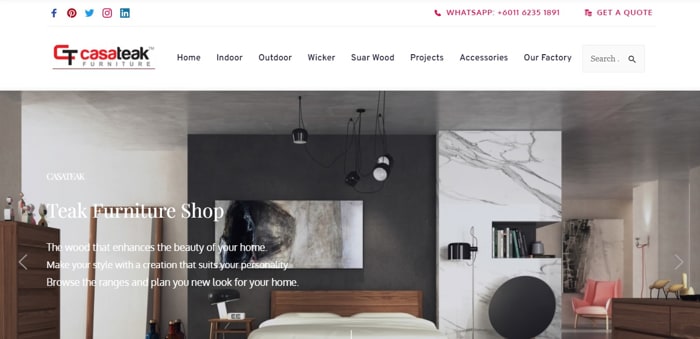A detailed screen capture from a website is depicted. At the top of the predominantly white page, various social media icons are displayed: the blue Facebook logo, the red and white Pinterest logo, the blue Twitter bird, the pink Instagram icon, and the white and teal LinkedIn icon. Towards the right side, written in red text, it says "WhatsApp: +6011-6235-1891" accompanied by a small phone icon. Below that, there's a prompt to "Get a Quote."

Further down, the webpage showcases "Casa Teak Furniture" in bold text alongside a black and red logo. The navigation menu includes sub-menus in black text: "Home," "Indoor," "Outdoor," "Wicker," "Sugarwood," "Projects," "Accessories," and "Our Factory." Adjacent to this is a grey search box with a grey magnifying glass icon inside it.

The main image boasts the phrase "Teak Furniture Shop" in white text over a white background, somewhat difficult to read due to the light backdrop. Beneath it, a tagline reads: "The wood that enhances the beauty of your home. Make your style with a creation that suits your personality. Browse the ranges and plan your new look for your home."

The image itself offers a glimpse into an aesthetically arranged room with various pieces of furniture and decor. In the foreground, a mirror is casually propped against a white wall, complemented by adjacent white ceilings. A brown dresser adorned with knickknacks sits nearby. To the right, a gray wall supports a black-and-white piece of artwork, while black pendant lights hang from the ceiling. Below this, a mid-tone brown headboard is paired with white bedding. A brown side table with a black lamp is situated next to it. 

In the lower section of the room, a gray and white marble-patterned object filled with books, a black lamp, and a black round object are visible. A pink chair contributes a pop of color, positioned beside a chocolate brown piece of furniture embellished with gold items. Behind the pink chair, another piece of black-and-white artwork is displayed, completing the room's sophisticated look.